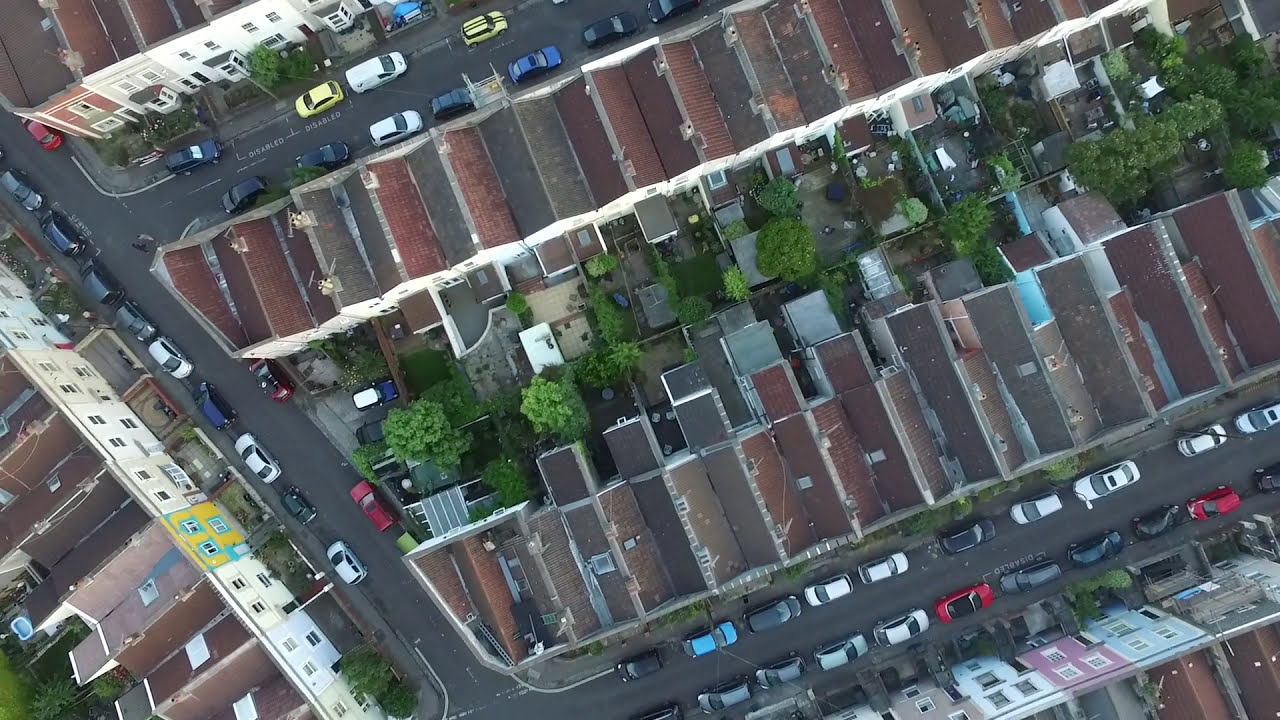This is a horizontal aerial image, captured from either a helicopter, airplane, or drone, showcasing a suburban neighborhood without tall buildings or skyscrapers. The image presents a densely packed residential area with two-story houses that are only two windows wide, positioned very close together. The houses are laid out in two distinct rows with additional houses on the periphery. Below the rows, we see varying colors of rooftops, all interconnected and extremely close to each other. 

Narrow streets run parallel and perpendicular to the rows, cluttered with bumper-to-bumper parked cars, allowing only a slim path for any moving vehicles. Behind the houses, there are small patios leading into communal green spaces featuring grass and trees, creating a shared outdoor area. The entire area has little more than 50 feet separating the rows of houses. The abundant trees scattered around further enhance the suburban aesthetic.